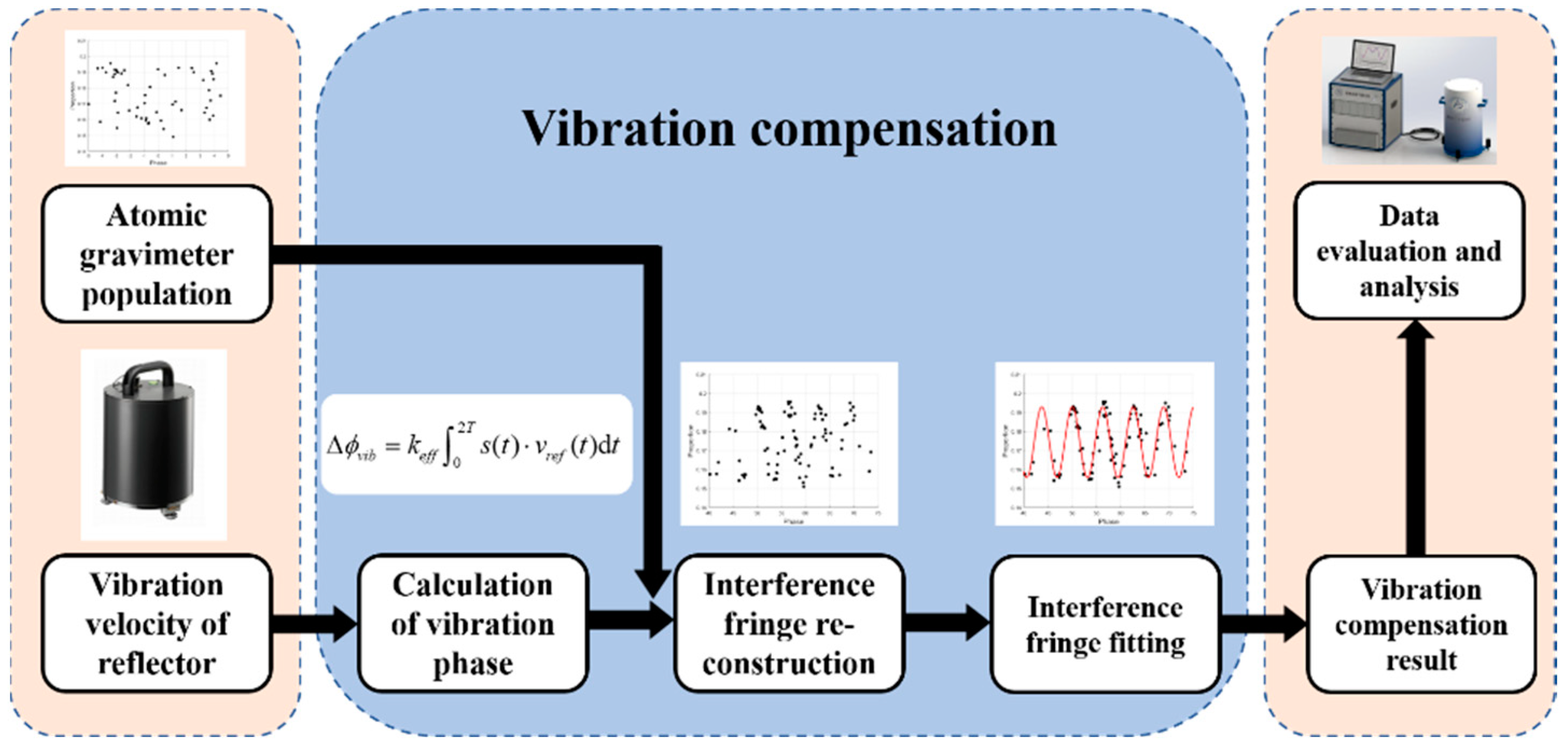The diagram is a flowchart detailing the process of vibration compensation, structured across three main sections. The central section is a large light blue rectangle with dotted rounded corners, titled "Vibration Compensation." On either side of it are tall cream-colored rectangles with rounded corners, representing different stages of the process.

In the cream-colored rectangle on the left, at the top, there is a graph followed by a white square labeled "Atomic Gravimeter Population," which has a black arrow pointing right and then downward to a black cylinder-shaped device below it. Further down, the square labeled "Vibration Velocity of Reflector" directs the flow into the central blue section.

Inside the blue rectangle, there are several interconnected boxes, each linked by arrows. The boxes are labeled "Calculation of Vibration Phase," "Interference Fringe Reconstruction," "Interference Fringe Fitting," and "Vibration Compensation Result," which are part of the vibration analysis sequence. The final stage in this blue rectangle is "Data Evaluation and Analysis," situated above the other boxes. Above this section, a photo depicts a square device with a blue frame connected to a two-toned (blue and white) cylindrical device by a wire.

Finally, the right cream-colored rectangle consolidates the results, including two charts below the title "Data Evaluation and Analysis." One chart has black dots in the middle, while the other features black dots alongside red lines going up and down, representing the analyzed data.

Overall, the diagram presents a comprehensive overview of the vibration compensation process from initial measurement through analysis, integrating visual aids, graphs, and device illustrations.